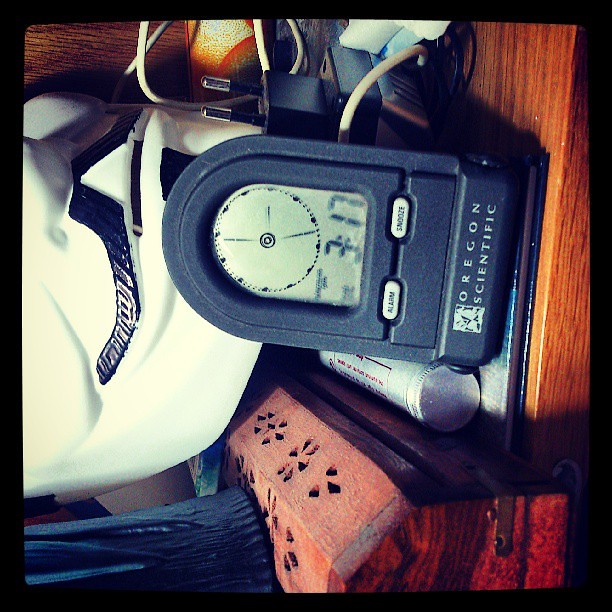The image features a variety of items and is of low resolution, presenting a somewhat grainy appearance. It appears to be oriented sideways, causing all elements to be tilted. Central to the image is a black-colored object, which is a digital device. This device prominently displays a digital screen and has "Oregon Scientific" written in white at its bottom.

Beneath the screen are two distinct buttons: the left button is labeled "Alarm" and the right button is labeled "Snooze." The digital display shows the time as 3:17 in black digits. Above the time display, additional details are partially visible but not completely discernible due to the image’s low quality and resolution.